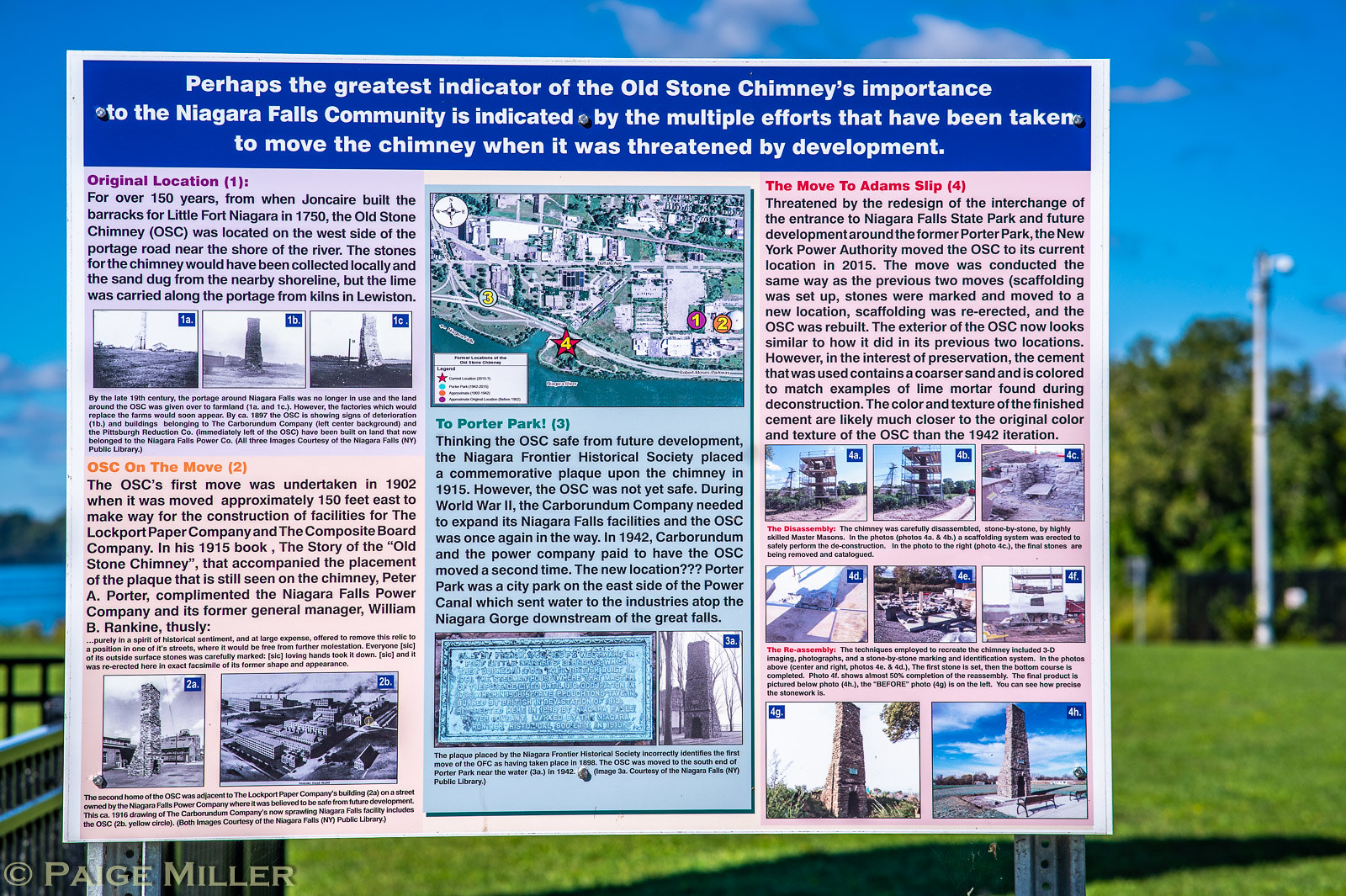This photograph captures a detailed billboard situated in a park, focused prominently against a blurred backdrop of green grass, leafy trees, and a hint of water. The sky is a bright blue, enhancing the outdoor ambiance. The billboard, supported by two metal posts, features a blue header with white typography highlighting "Old Stone Chimney" and its significance to the Niagara Falls community. The text commends the community’s dedication, evident in the multiple relocations of the chimney to protect it from development threats. Notably, the billboard is adorned with various drawings, architectural designs, and photographs. It narrates the chimney's journey through its original location, subsequent moves indicated by the title "OSC on the Move," relocation to Porter Park, and eventually to Adams Slip. At the bottom left-hand corner, the sign credits copyright to Paige Miller. The narrative is visually organized with columns and color-coded sections, emphasizing the chimney's historical and cultural value by chronicling its relocations and reassembly near the current park.